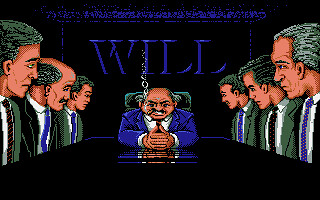This is a computer-generated image that resembles a scene from a video game. The picture is small and has a rectangular, panoramic orientation, emphasizing its wide perspective. At the center of the image sits a Caucasian CEO, dressed in a blue suit, a white shirt, and a red tie. He has his hands entwined together on a long black table, and a cigar dangles from his mouth, with smoke visibly trailing upward. His image and shadow are both reflected on the glossy surface of the table, adding depth to the scene.

Surrounding the CEO at the table are six men, three on each side. On the left side, the middle individual is bald, distinguishing him from the others. Most of these men are wearing green suits, while the remaining few are dressed in black suits. Their neckties vary in color and pattern; some are blue, some have polka dots, and one particular tie stands out with its black base and orange stripes.

The backdrop is stark black, which contrasts sharply with the bright blue letters "WILL" displayed in all capitals. Above this word is a blue stripe, and on either side, two thin blue lines frame the word, adding a minimalistic yet striking element to the overall composition.